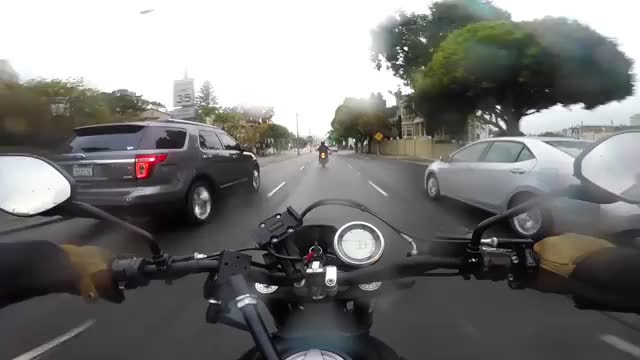The image is an outdoor, daytime photograph captured during rain, evidenced by the hazy raindrops on the camera lens. Taken from the point of view of a person riding a motorcycle, likely with a GoPro-style camera, the foreground prominently features the motorcycle's black handlebars, on which a pair of hands wearing tan gloves and a black coat are gripping. The rearview mirrors on either side of the handlebars are visible with their round reflective surfaces. The rider is in the middle lane of a three-lane road marked by white dotted lines. Ahead, another dark-colored motorcycle is visible, situated two or three car lengths away. Flanking the rider's motorcycle, there is a gray SUV on the left and a silver four-door sedan on the right, all moving in the same direction. The scene is lined with green trees on both sides of the road. Additionally, there are some buildings on the sides and a speed limit sign indicating 35 miles per hour is visible. The overall atmosphere is overcast, with gray skies hinting at recent or ongoing rain.